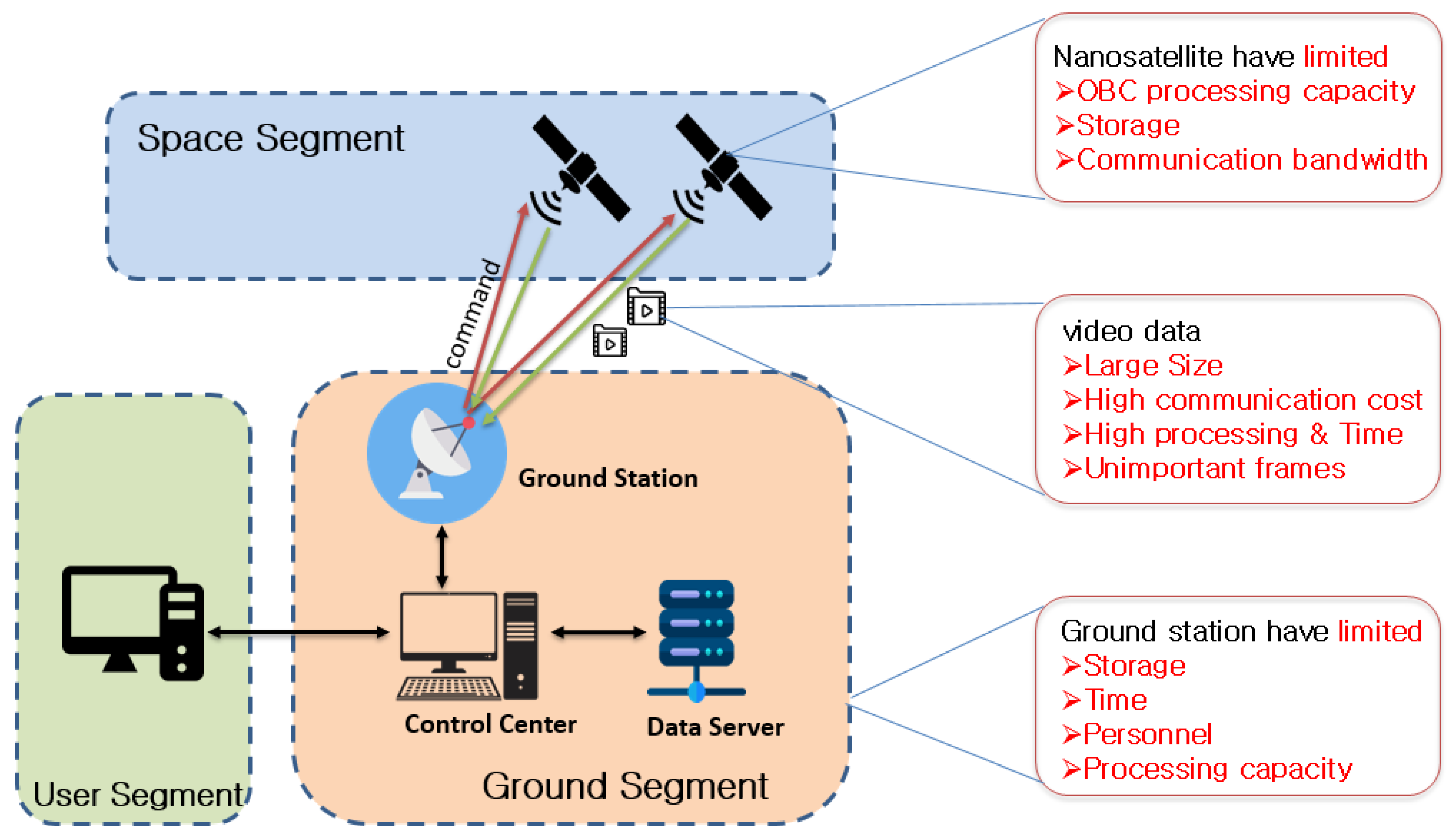This infographic illustrates the communication network of electronic components involved in satellite data transmission. At the top of the white background image, a light blue, horizontally oriented rectangle labeled "Space Segment" is outlined with a dashed black line. Inside this rectangle are two black icons representing satellites emitting radio waves. Below and to the left, a light green, vertically oriented rectangle labeled "User Segment" features an image of a computer monitor and a black remote control. Adjacent to this, a tan square labeled "Ground Segment" is also bordered by a black dashed line. Within this box, the upper left corner showcases a white radar inside a blue circle labeled "Control Center," depicting a computer monitor and CPU setup below it. To the right, various pieces of electronic equipment, labeled "Data Server," highlight the data flow. Additional boxes to the right provide textual details such as the limitations of nanosatellites, including processing capacity, storage, and communication bandwidth, alongside notes on video data size and ground station constraints like limited storage, time, personnel, and processing capacity. Red and green arrows indicate the bidirectional flow of information between the ground station and satellites, underscoring the interconnectedness of these segments in coordinating satellite data for internet usage.